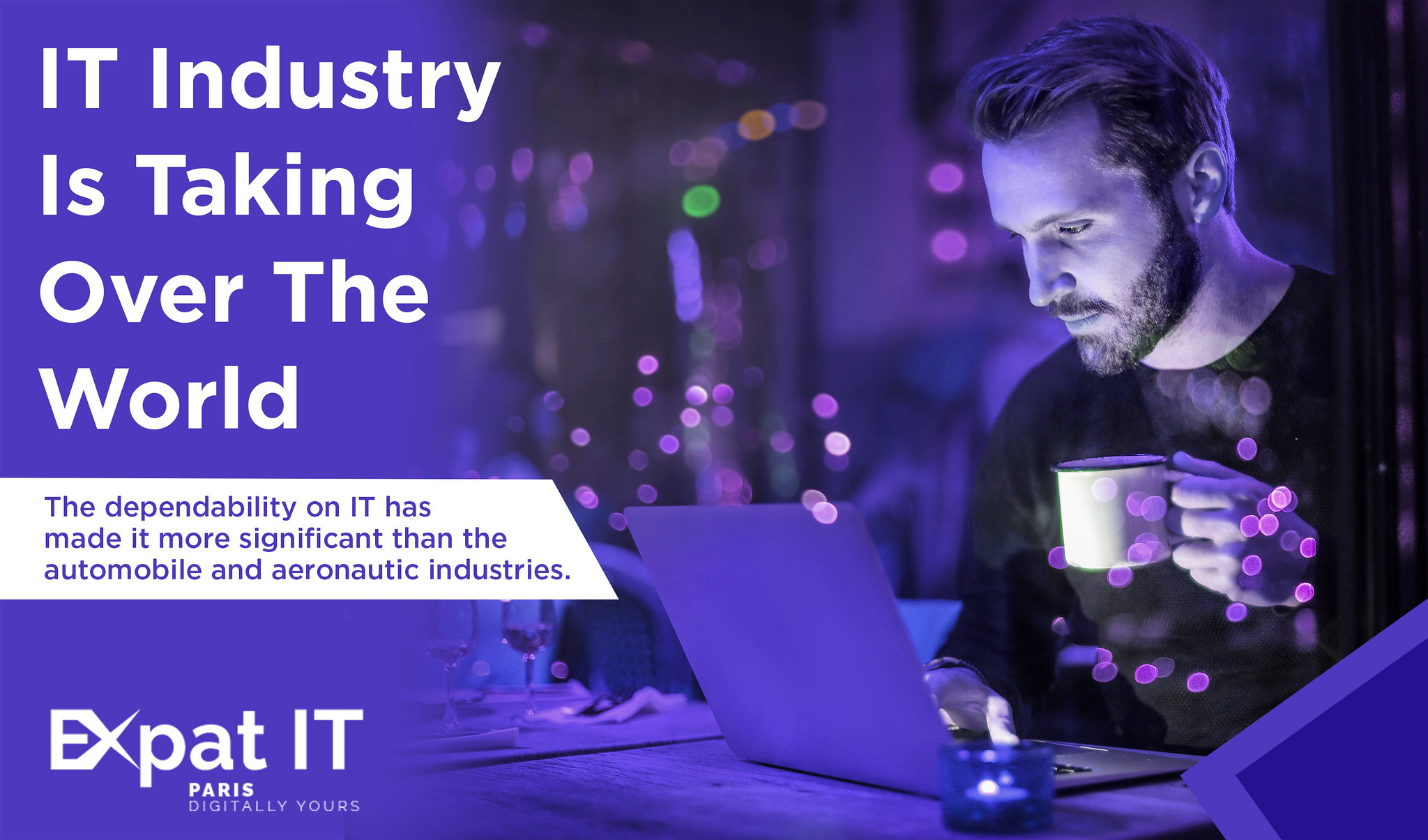This image appears to be an advertisement predominantly featuring shades of purple, black, and white. On the right side, there is a man seated at a desk, illuminated by a soft light emanating from his laptop. He has a short beard and mustache, and he is dressed in a long-sleeved shirt. The man is holding a white coffee mug in his right hand while tapping on his laptop with the same hand. His workspace includes a variety of items, such as a wine glass, a candle, and some silverware, adding to the cozy yet professional ambiance. Surrounding him are twinkling lights that enhance the warm atmosphere. The left side of the image features a purple overlay with white text stating, "IT industry is taking over the world." Below this, in purple text on a white background, it reads, "The dependability on IT has made it more significant than the automobile and aeronautic industries." Further down, in white text again, it states, "Expat IT, Paris, digitally yours." Scattered across the image are clusters of pink dots, accentuating the design.